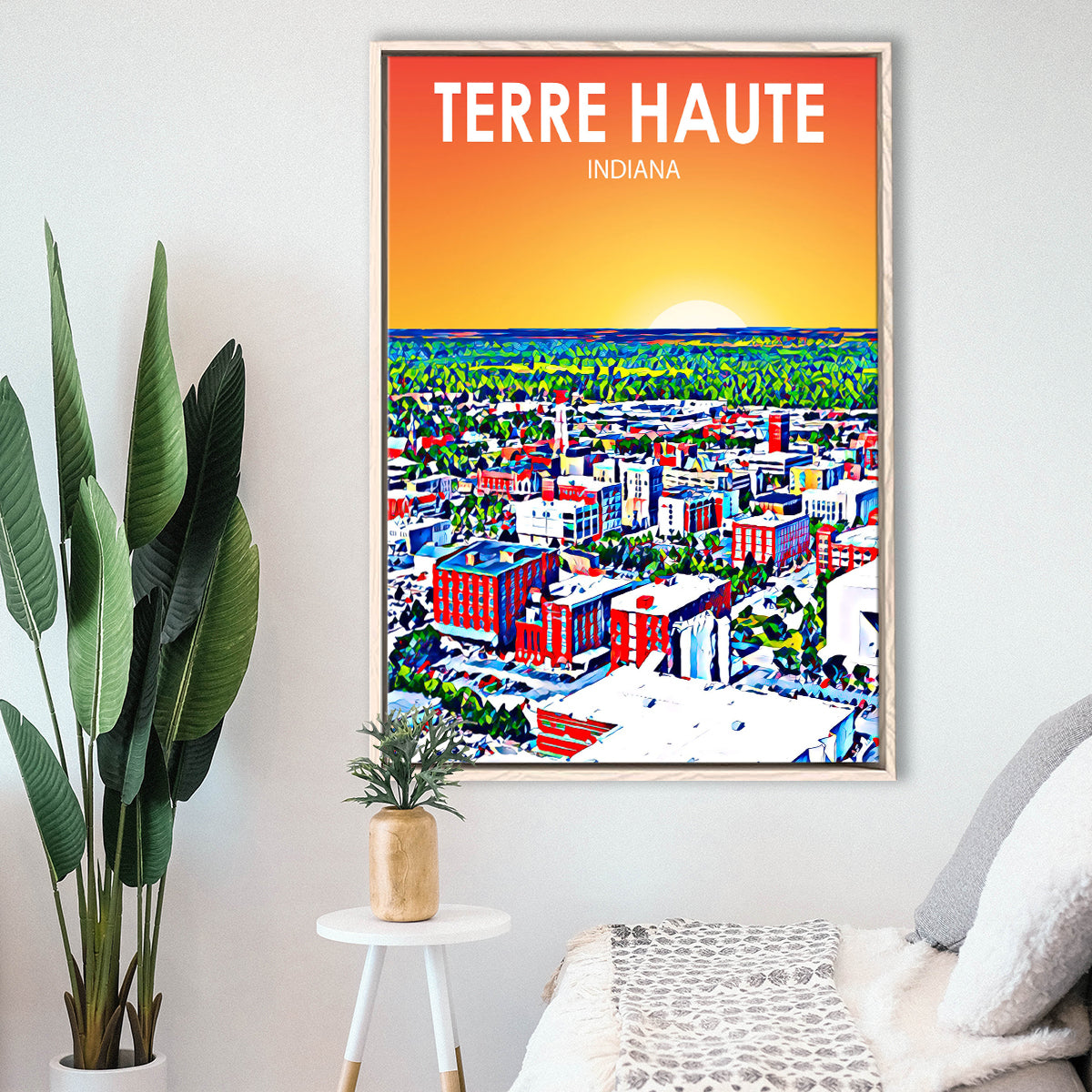This photograph showcases a room with a minimalist aesthetic, characterized by white walls and accented by thoughtfully chosen decor. Dominating the wall is a large, Art Deco-style poster of Terre Haute, Indiana, which features vibrant hues of orange, yellow, blue, green, white, and red. The scene depicted in the poster includes various buildings in the foreground and a horizon with crops and a sun setting in the distance, evoking a modernistic cityscape.

In the bottom left corner of the room stands a substantial floor plant with large, elongated leaves, its narrow vase lending height to its stature. Adjacent to this tall plant is a three-legged white stool serving as a table, which holds a smaller plant nestled in a golden holder. To the right, a cozy white couch or day bed is adorned with a fuzzy white blanket, a gray and white runner, and two pillows—one fuzzy white and the other gray—adding layers of texture and comfort to the seating area. The thoughtful arrangement of furniture and decor elements creates a harmonious and serene atmosphere within the room.